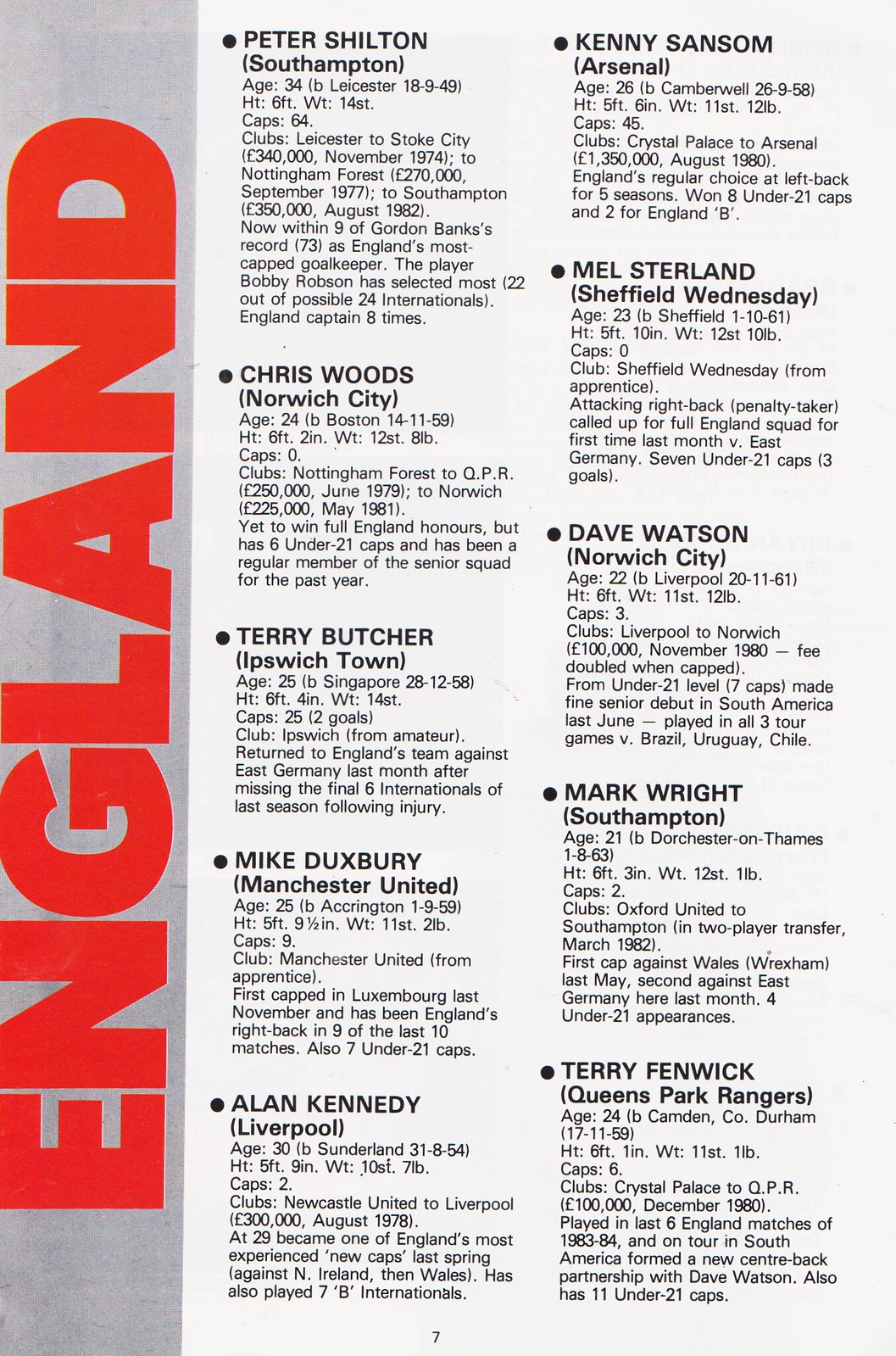The image appears to be a scanned magazine page, prominently featuring a vertical grey band on the left side with the word "England" in large, bold, red text running vertically. To the right, there's a light blue background showcasing a detailed bullet list of names, presumably soccer players, organized into two columns. This list includes information such as the players' names, current teams, and various statistics, such as age, height, and clubs they've played for. The left column includes Peter Shilton (Southampton), Chris Woods (Norwich City), Terry Butcher (Ipswich Town), Mike Duxbury (Manchester United), and Alan Kennedy (Liverpool). The right column features Kenny Sansom (Arsenal), Mel Sterland (Sheffield Wednesday), Dave Watson (Norwich City), Mark Wright (Southampton), and Terry Fenwick (Queen's Park Rangers). Each name is accompanied by further detailed stats like age, height, weight, caps, club history, and playing position.